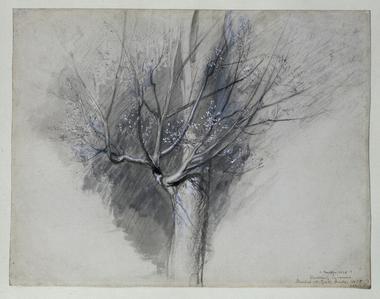The image is a detailed hand-sketched artwork of a tree, depicted using what appears to be pencil or charcoal on a grayish paper background. Positioned centrally within a small, square frame, the narrow tree trunk extends upward to the top of the image. Emanating from the tree's midsection is a prominent branch that stretches out, with numerous slender twigs branching off in various directions.

These twigs are adorned with very small flower petals or tiny leaves. The background behind the tree is subtly shaded, adding depth to the composition. At the bottom right of the artwork, there is a faint, unreadable signature or some form of writing, further adding to the artistic presentation. The entire image is rendered in monochrome, utilizing shades of white, black, and gray. The setting and style suggest it might be an art class project or an artist's portfolio piece.